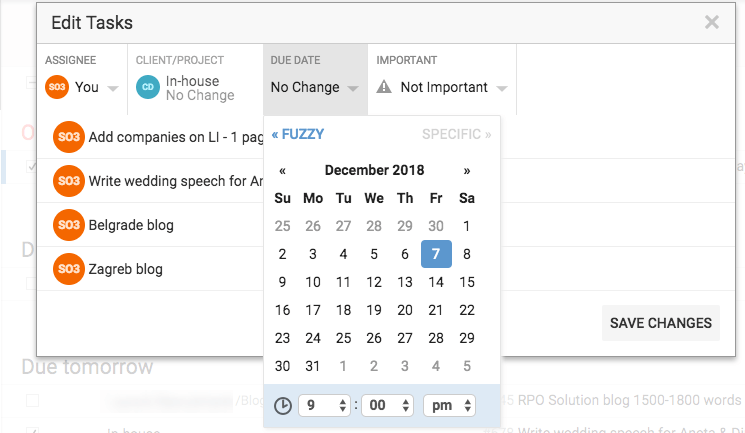This horizontal image, likely viewed on a smart device or computer, features a layered interface commonly seen in task management or productivity software. In the background box, partially obscured by an overlay, there's a checklist item with a checkmark and a border. The visible text reads "Due Tomorrow" followed by "RPO solution blog" with a word count range of "1,500-1,800 words." 

Overlaid atop this background is a black task-editing box labeled "Edit Tasks" with a gray X button in the upper right corner to close it. On the left, there's a section titled "Assignee" displaying several orange-circled tasks assigned to various entities like "You," "Add Companies," "Write Wedding Speech," "Belgrade Blog," and "Zagreb Blog," all marked with an SO3 tag.

To the right of the assignee section, there's a "Client Project" field marked by a seafoam green teal circle with the label "CD in-house no change." Below, the due date section reads "Fuzzy or Specific," with "Specific" highlighted in blue, showing "December 2018, Friday the 7th at 9 p.m."

There is also an "Important" section featuring a triangle with an exclamation point and a label that toggles between "Not Important" and "Important." At the bottom right of the overlay, a "Save Changes" button is visible, allowing the user to finalize their task edits.